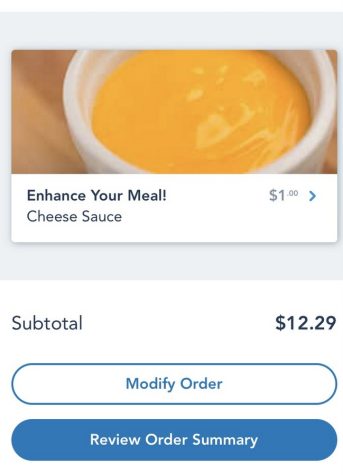The image displays a clean and minimalist mobile user interface for a food ordering app. At the top, there's an option to enhance your meal with cheese sauce priced at $1. This option is accompanied by a subtle drop shadow and includes an image of a small ramekin filled with cheese sauce placed on a wooden cutting board or table. Below this menu option, the subtotal is listed as $12.29.

Beneath the subtotal, there are two prominently placed blue buttons: "Modify Order" and "Review Order Summary." These buttons are designed with rounded corners, making them visually appealing and easy to interact with. The entire setup is devoid of any extraneous information, such as a taskbar or phone details, suggesting the image has been cropped. The background is a plain white, enhancing the clean and focused aesthetic of the interface. Overall, the user interface is both functional and visually pleasing.